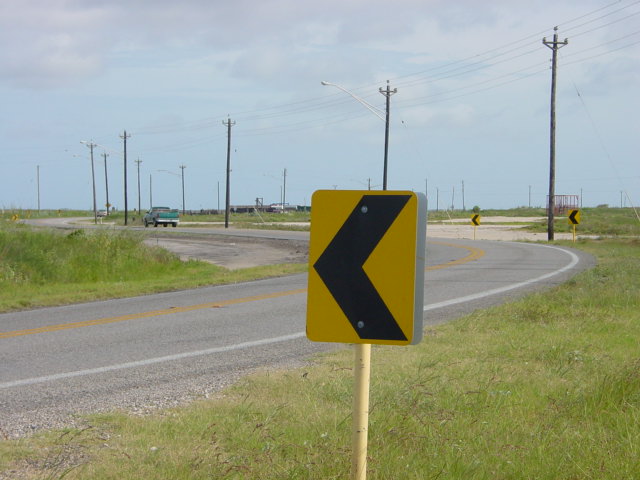The photograph depicts a winding, two-lane road stretching into the distance under a bright blue sky scattered with white clouds. The road, which is gray with yellow lines down the center and white lines along its edges, begins in the bottom left corner, curves to the left, and then takes another right curve further along. There are multiple signs along the road—yellow rectangles with black left-pointing arrows—on both sides, particularly around the curves, mounted on steel and wooden poles. 

A blue car is positioned near the left side, approaching the second right curve, while a green van with a white stripe is further ahead. Grasslines the sides of the road, varying in length from short near the road to longer farther away. Power lines run parallel to the road, attached to black poles, with a white light illuminating the second pole from the right. The flat landscape extends with no hills in sight, featuring elements of an industrial area with visible steel structures in the background.